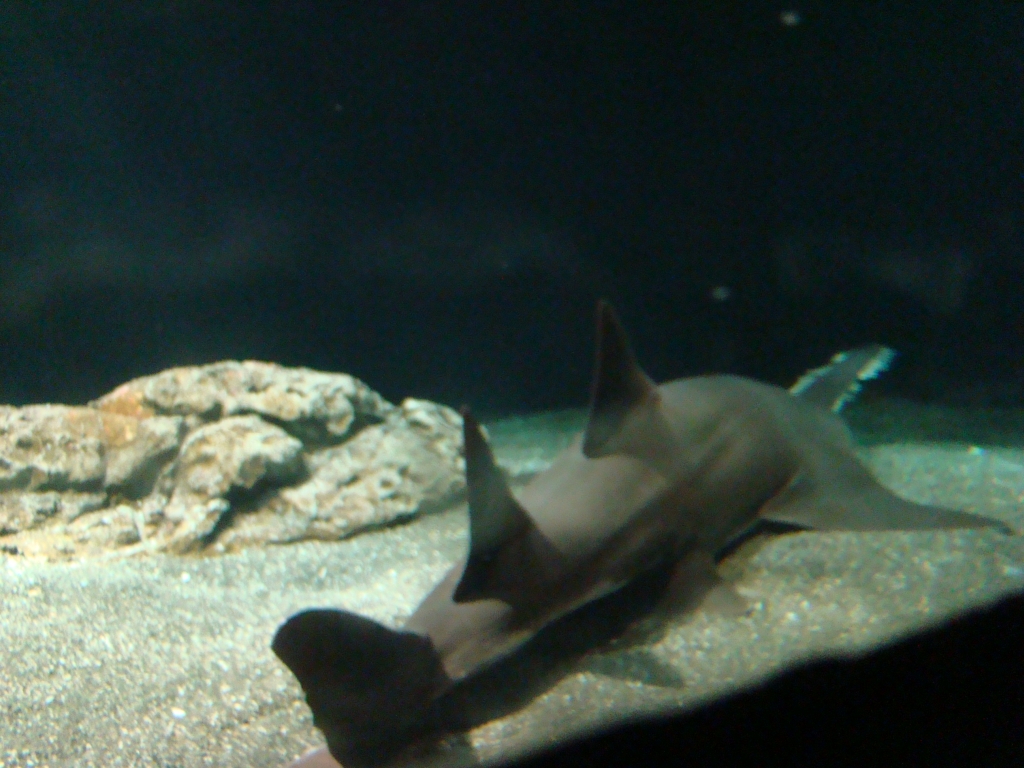This image presents an underwater scene, likely captured within an aquarium due to the distinct artificial boundaries suggested by the consistent light brown substrate and the abrupt end of the ground at the edge of the frame. The backdrop is a deep black, enhancing the focus on the foreground elements. A brownish-beige rock, featuring a subtle copper spot, sits prominently on the sandy bottom, which appears coarse and free of algae, suggesting a well-maintained environment.

Dominating the scene is an intriguing fish, resembling a hybrid between a shark and a manta ray. Its body features a pair of dorsal fins and a typical shark tail, yet it extends into side fins akin to those of a manta ray. The fish’s front is characterized by a sword-like protrusion. The animal is moving diagonally, approximately toward the one o'clock direction from the image's center. Notably, shadows of the fish's fins are visible on the sandy substrate, adding depth and dimension to the composition.